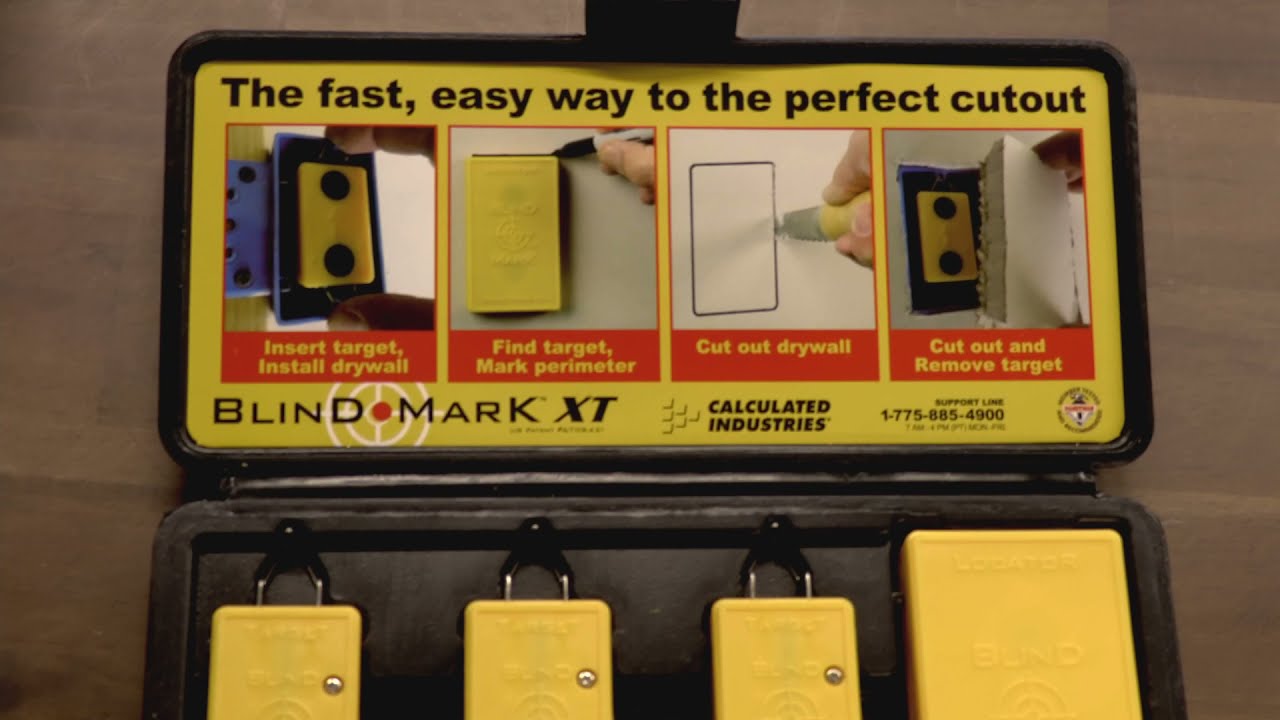The image shows an open black plastic case containing a toolkit designed for making precise cutouts in drywall to locate electrical boxes. The inside lid of the case features a bright yellow background with black text that reads "The fast, easy way to the perfect cutout." Below this text are four instructional photographs arranged from left to right, each illustrating a step in the process: inserting a target and installing drywall, marking the perimeter of the target with a marker, cutting out the drywall along the marked lines, and finally removing the cut piece. Under these images, black lettering spells out "Blind Mark XT" alongside a logo for the manufacturer, Calculated Industries, and a support line phone number: 1-775-885-4900. In the main compartment of the case below these instructions, there are several bright yellow rectangular locator devices, each with silver rings at the top. The entire case rests on a brown surface, possibly a wooden floor.